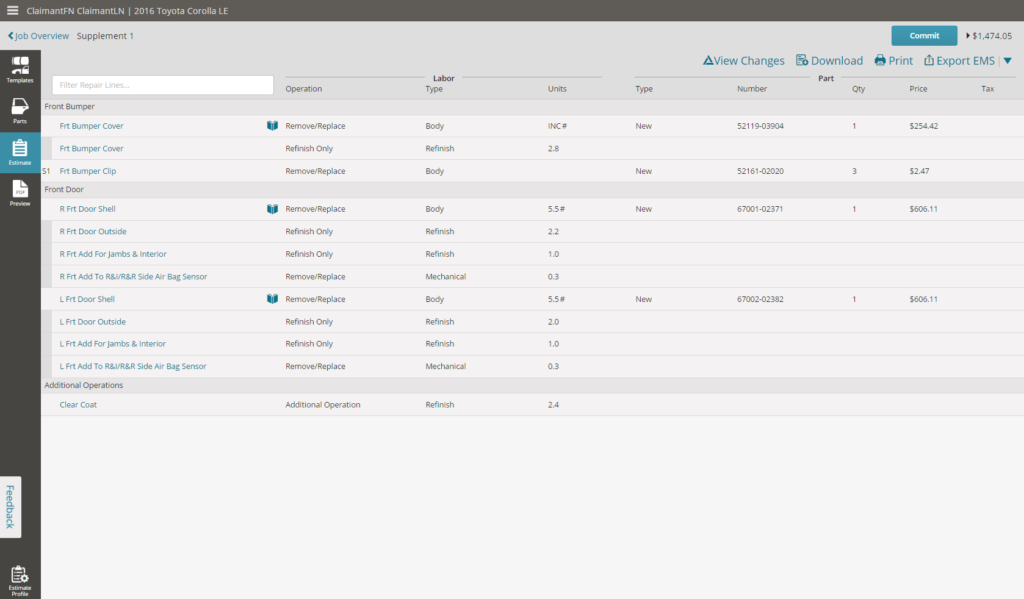The web page features a predominantly light gray and light purple background, accented by a thin black ribbon running horizontally across the very top of the screen. On the top left corner, there are three horizontal bars, followed by the text "Claimant FN" and "2016 Toyota Corolla LE," indicating the subject and model of the auto repair estimate.

Beneath this header, set against a darker gray background, the words "Job Overview" are prominently displayed in bright blue. To the left of this title is a back button, and to its right, in gray text, is "Supplement One." This section clearly marks the page as an estimate for auto repairs for the specified Toyota Corolla LE.

On the very top of the page is a search box. The content of the estimate is divided into two primary categories: "Labor" and "Parts," with a vertical list of detailed information under each category. A black ribbon runs vertically down the left-hand side of the screen. At the top of this ribbon is the template icon labeled "Templates." Directly below it is the "Parts" section, marked with a car door icon. The "Estimates" section is highlighted and features a clipboard icon. Finally, the "Preview" option, which displays a PDF document, is located at the bottom of this vertical menu.